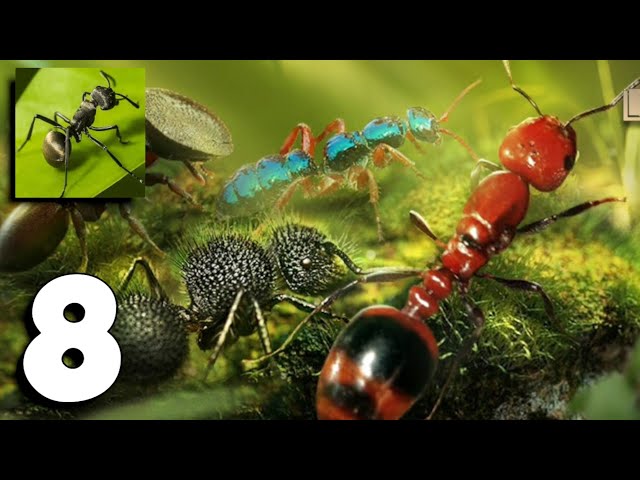This detailed, close-up image features four distinct types of ants, all navigating a lush, green patch of grass. Dominating the right-hand side, the largest ant is vividly red with striking black and red stripes on its thorax. Nearby, a dark gray, spiky ant composed of three segmented parts stands out, with a metallic sheen that catches the light. Slightly in the background, an iridescent blue ant with reddish-orange legs and antennae adds a colorful contrast. Additionally, a partially visible brown ant appears beneath a smaller, typical black ant perched on a green leaf in the top left corner. The image is bordered in black along the top and bottom edges, with a bold, cartoony white number eight prominently displayed in the bottom left corner.